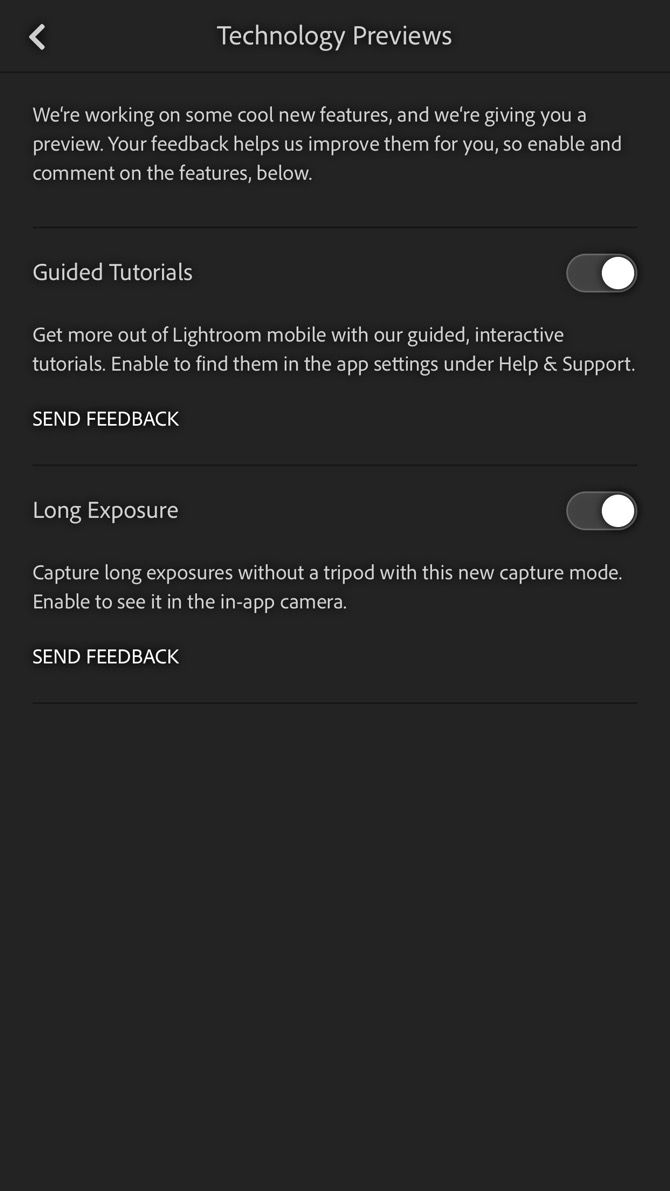The image depicts a website interface with a sleek, completely black background. Prominently displayed at the top is the title "Technology Previews," followed by a brief introduction stating, "We're working on some cool new features and we're giving you a preview. Your feedback helps us improve them for you, so enable and comment on the features below."

Below the introduction, the first preview feature listed is "Guided Tutorials." Accompanying this feature is a toggle switch, currently set to the off position. The description for this feature reads: "Get more out of Lightroom Mobile with our guided interactive tutorials. Enable to find them in the app settings under Help & Support."

Following that is another section titled "Send Feedback," focused on a feature called "Long Exposure." This feature also has a toggle switch in the off position and includes the description: "Capture long exposures without a tripod with this new capture mode. Enable to see it in the in-app camera." Beneath this description, in all uppercase and white text, is a call to action: "SEND FEEDBACK."

From this point down to the bottom, the image shows a continuous black box, suggesting a minimalist design. Based on the vertical orientation and the dimensions of the image, it appears as though this interface could be displayed on a mobile device. However, no specific phone icons are visible at the top to definitively confirm this.